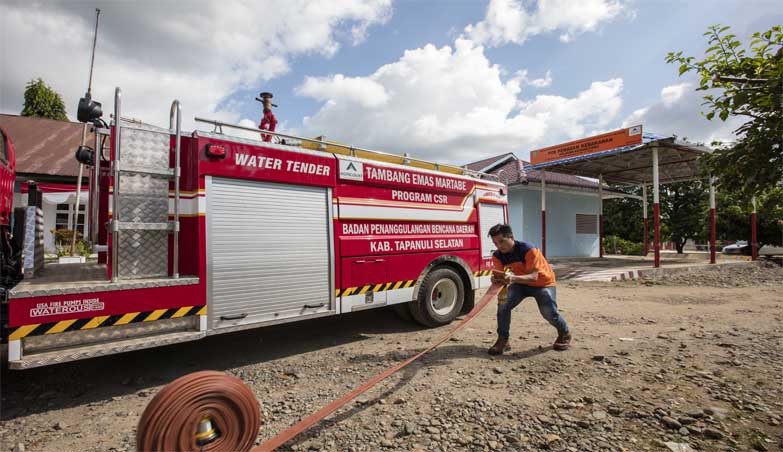In the photograph, a man in his 30s or 40s with dark hair, dressed in an orange shirt and jeans, is prominently featured in the center. He is rolling up a rust-colored fire hose. To the left of him stands a red and white fire truck, with a silver door that lifts up and a metal ladder. The truck is marked with various texts such as "Water Tender," "TAMBAG EMAS," "MARTABE PROGRAM CSR," and "BADAN PENANG GULANGAN BENGAL CAB TAPANULI SALADAN." The vehicle is cut off at the front, revealing its side view. The scene is set on a dirt and rocky ground, with an abandoned white building with boarded-up windows and a blue roof in the background. Further behind, there are a few cars and many trees. The sky above is blue, dotted with white and some gray clouds, creating a picturesque backdrop.